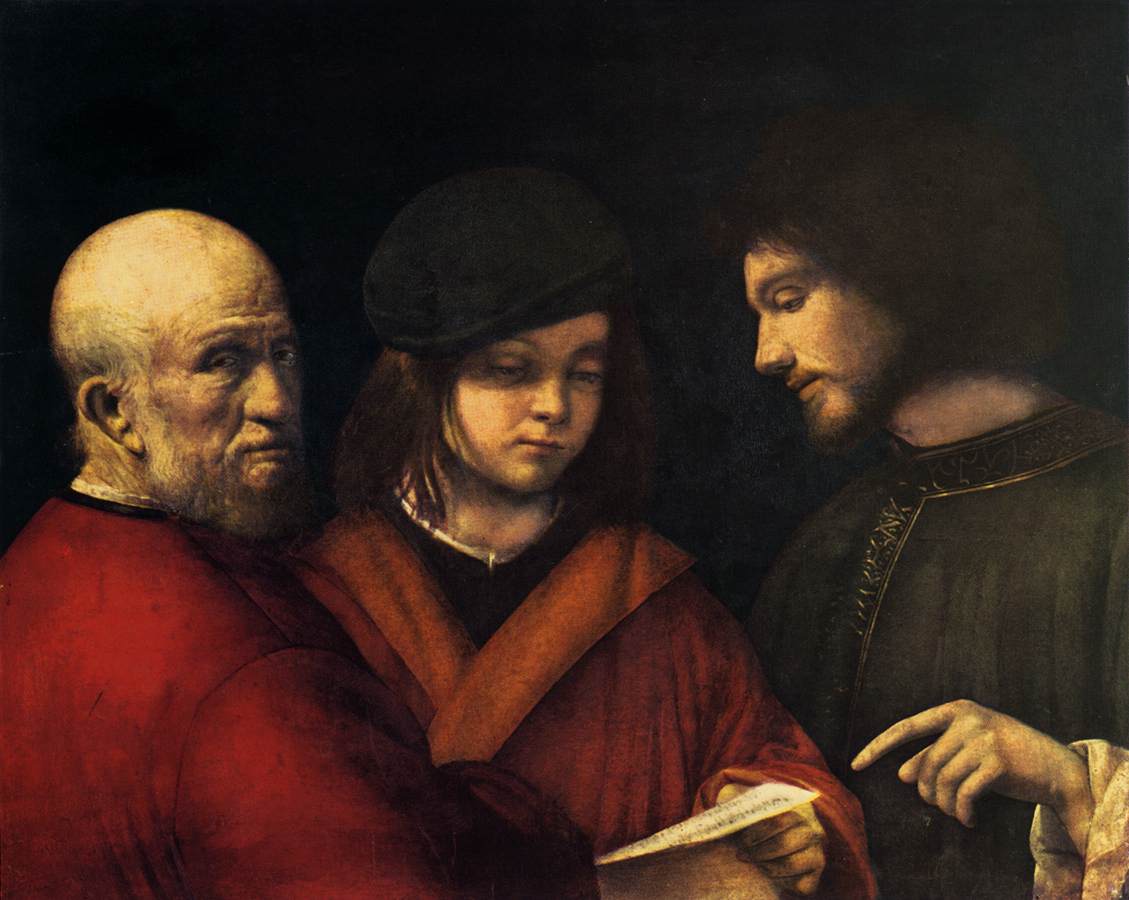The painting depicts a somber, medieval scene featuring three people against a completely black background. On the left is an old, bald man with a beard, dressed in a red coat. His body is angled towards the center figure, but he gazes directly at the viewer. The central figure is a young person with shoulder-length brown hair, wearing a distinct black beret and an orange quilted robe. This young individual appears to be around fourteen years old and holds a piece of paper in their left hand, their expression neutral and introspective. To the right, there is another man with long hair and a slight beard, clad in a dark gray robe. He focuses intently on the piece of paper, pointing at it with his left hand. The overall mood conveyed by their expressions is one of subtle sadness or contemplation.